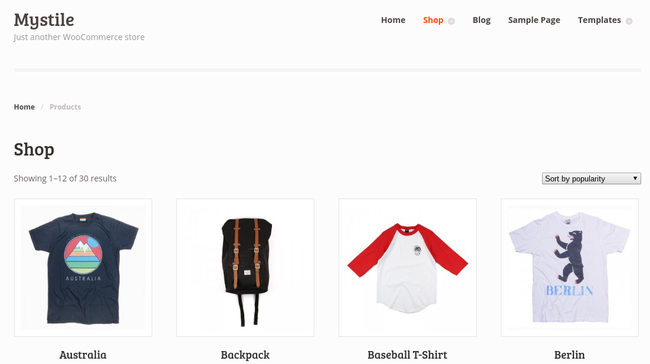**Detailed Caption:**

The image appears to be a screenshot of a shopping page on a website called MyStile, which is a WooCommerce site. The background is solid white with a hint of off-white gray, giving it a subtly textured look. A barely visible border surrounds the entire screen, blending seamlessly with the background.

In the upper-right corner of the website, the header displays the site's name, "MyStile," in bold text, followed by the tagline "Just another WooCommerce site" in smaller, regular text beneath it. Below the header, there is a navigation bar with clickable sections labeled: Home, Shop, Blog, Sample Page, and Templates. The Shop section is highlighted in orange, indicating the current active page.

Directly below the navigation bar is a thin gray border and a breadcrumb trail that reads 'Home / Products' with 'Home' in bold text. Below this, the page indicates it is showing "1 of 12 of 30 results." On the far-right side of this section, there is a sort button currently set to "Sort by popularity," presented within a gray text box.

The main content of the page features a grid of product listings. The first item, displayed on the far left, is a black t-shirt featuring a mountain graphic and labeled "Australia." It is showcased within a white square box. Next to it is a black backpack with gray straps, also within a white square box. The third product is a white baseball t-shirt with red mid-length sleeves. The last item on the far right is a white t-shirt that has "Berlin" printed in blue, accompanied by an image of a bear facing left above the text. Each product is neatly displayed, giving a clear view of its design and features.